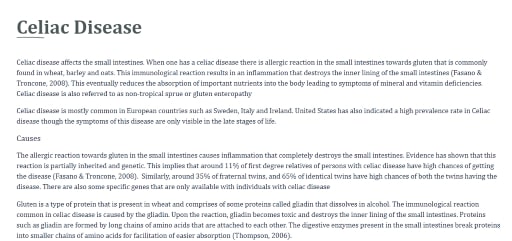A blurry screenshot providing information about celiac disease is displayed. The image features four different paragraphs, all written in gray text against a white background, with the heading "Celiac Disease" underlined at the top. Despite the poor quality of the screenshot, some content can be discerned. The text explains that celiac disease affects the small intestines, triggering an allergic reaction to gluten—an ingredient found in wheat, barley, and oats. This immunological reaction causes inflammation that damages the inner lining of the small intestines, leading to reduced absorption of essential nutrients and resulting in symptoms related to mineral and vitamin deficiencies. The condition is also known as non-tropical sprue or gluten enteropathy. It is more prevalent in European countries like Sweden, Italy, and Ireland, and is also increasingly common in the United States, where symptoms typically appear later in life. The image also contains two additional paragraphs discussing the causes of celiac disease, although these sections remain indistinct due to the blurriness.